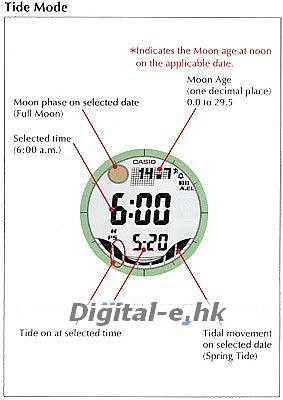This image features a detailed, diagrammatic clock face that highlights various elements related to time, moon phases, and tidal movements. At the center of the clock, the selected time is prominently displayed as 6:00 a.m. To the left of the clock face, an explanatory diagram delineates the significance of each component. Specifically, the 6:00 a.m. time is labeled as the selected time. Above the clock, an illustration of the moon indicates it represents the moon phase on the selected date, noting that it is a full moon. Additionally, at the very top, there is a legend explaining that the moon age at noon on the applicable date is displayed, with the age ranging from 0.0 to 29.5 days. At the bottom of the image, the brand name "Digital-E, HK" is clearly marked. Below this, information about tidal movements is provided, stating that it is a spring tide at the selected time. The entire diagram is titled "Tide Mode" at the top, encapsulating the image's function of conveying complex temporal, lunar, and tidal information.